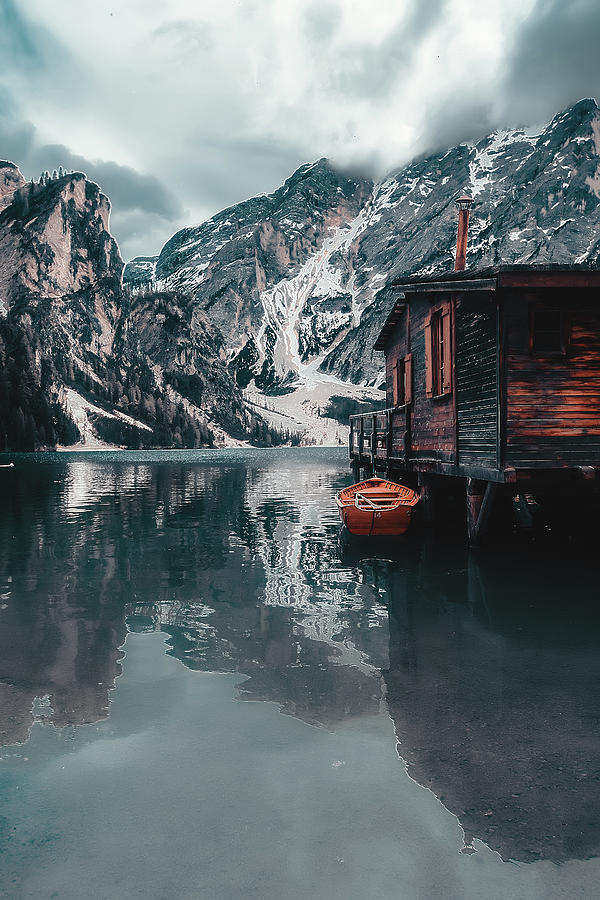The image captures a serene lakeside scene under a mostly cloudy sky. The calm, blue water fills the lower half of the frame, reflecting the rugged, snow-dappled mountains and gray clouds above. Dominating the right side of the image, a partially cropped wooden lake house stands elevated on high beams or stilts. Painted in warm shades of orange with black accents, the building features several windows and a railing, giving it a distinct yet rustic appearance. Attached to it is a small rowboat, moored close to the base of the elevated structure. The mountains in the background, with their rocky faces and patches of snow or perhaps water streams, add a majestic backdrop to this idyllic, almost painting-like scene.